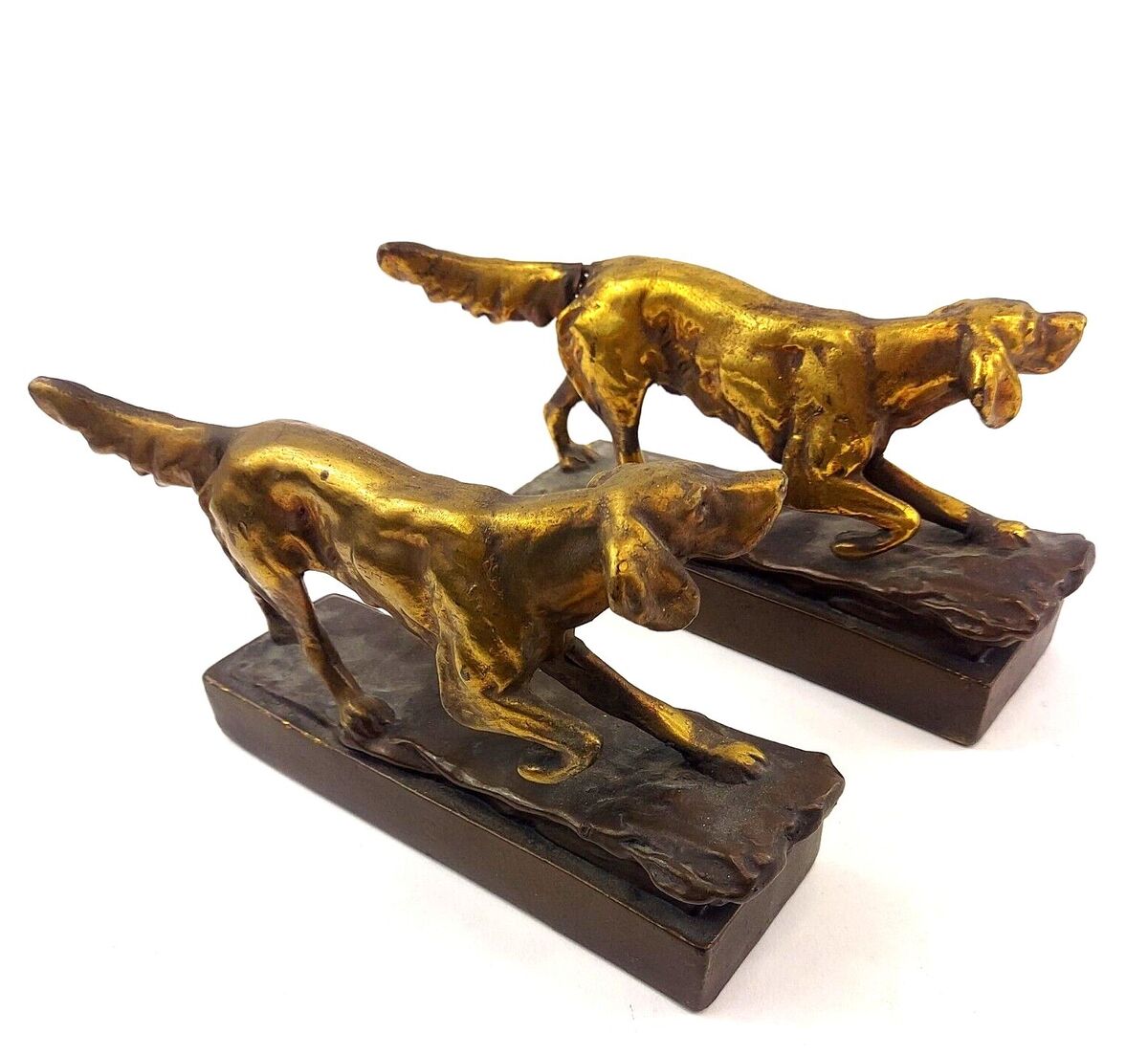The image depicts two gold statues of hunting dogs with wide ears and bushy tails. Each dog is in a crouching position, looking alert as if sniffing something, with its ears flopped down and tail stretched outward. Both statues are positioned side by side and facing towards the upper left portion of the screen, creating a parallel alignment from the top left to the bottom right. The dogs' stances are almost identical, with the left paw extended forward and the right paw slightly tucked in, while their two back paws remain grounded on textured bases that resemble logs but appear to be fashioned from dark brown material. Notably, the second statue is slightly shinier than the first, though both share the same intricate design. The background is pure white, emphasizing the detailed and lifelike features of the statues.